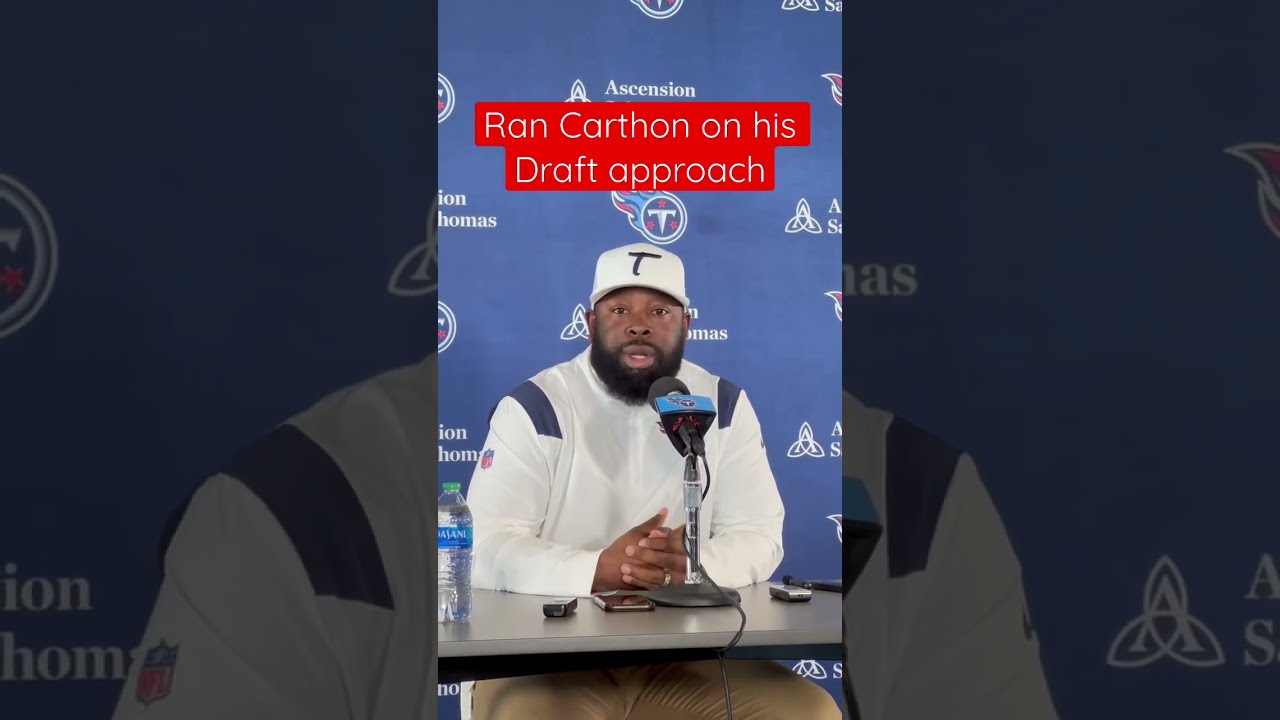In the image, an African-American man, identified as Ran Carthon, is captured during a press briefing. He sports a thick, medium-length beard and dons a white baseball cap emblazoned with the letter "T". His attire includes a white windbreaker-style jacket featuring dark blue shoulder accents and an NFL logo on the right sleeve. At the table, where a bottle of water is placed to his left, Carthon's hands are folded, showcasing a ring on one finger. The setting appears to be a sports-related event, possibly a post-game press conference, as suggested by the blue step-and-repeat banner behind him adorned with staggered logos and the word "ascension" printed repeatedly. Overhead, a red text box with white lettering prominently displays, "Ran Carthon on his draft approach."